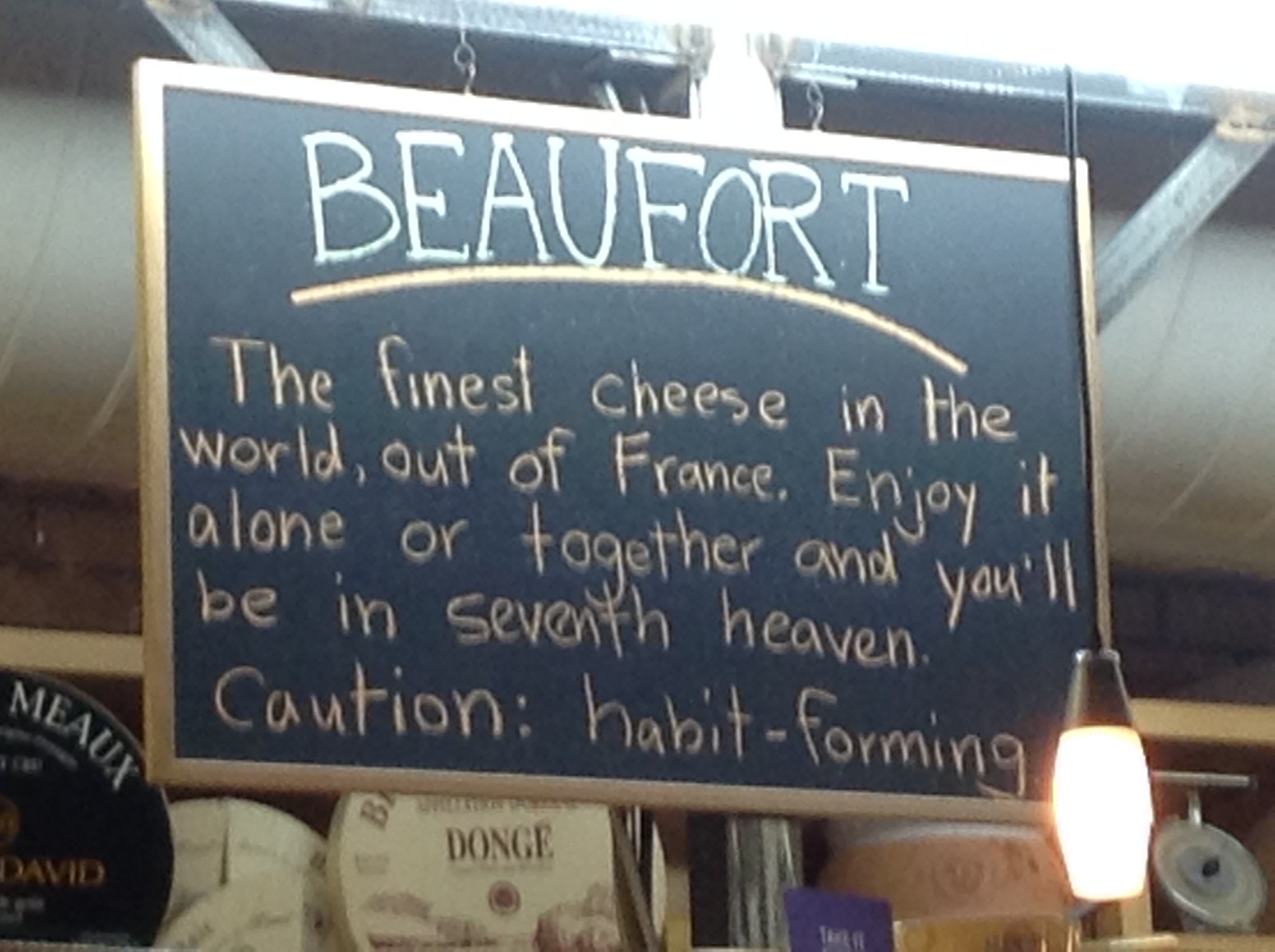The image depicts a chalkboard sign with a wooden border, hanging from the ceiling of a restaurant or grocery store. The sign itself is a blackboard with text written in chalk. At the top, in large white capital letters and underlined in orange, it reads "Beaufort." Below this, in orange chalk, is the phrase "The finest cheese in the world, out of France. Enjoy it alone or together, and you'll be in seventh heaven." A cautionary note below states, "Caution, habit forming."

Adjacent to the sign, there is a pendant light hanging from a thin black wire, illuminating the area. Beneath the chalkboard, a shelf displays several wheels of cheese, each with distinct branding. Notable among them are a cream-colored wheel labeled "Dongé" and another wheel marked with "Meaux" in white lettering on blue packaging. This charming setup emphasizes the variety of high-quality cheeses available for purchase.